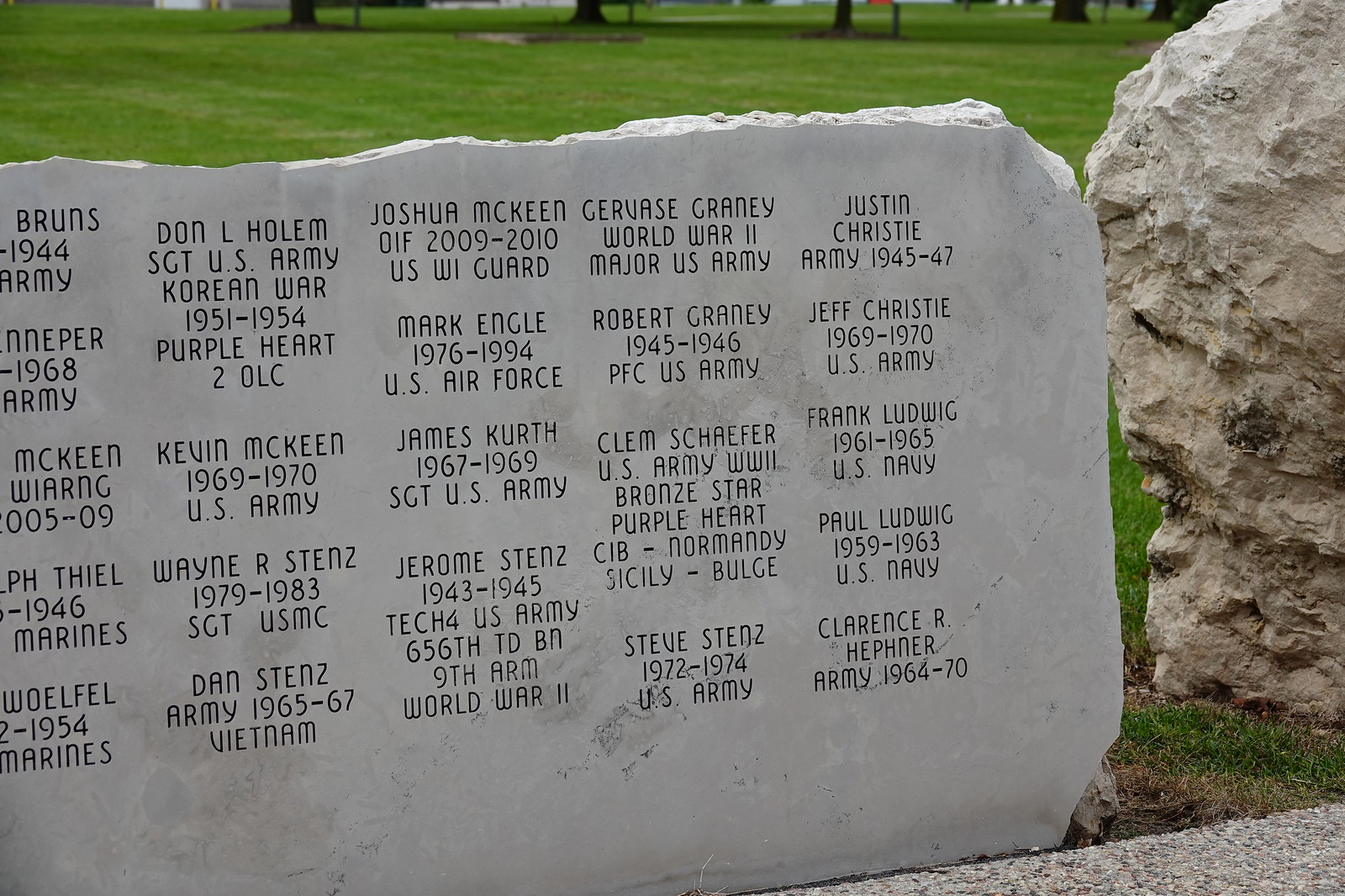The image depicts an outdoor memorial site featuring a large, engraved slab of white marble prominently displayed on the left side and extending towards the center. To the right of the marble slab, there is a smaller gray and brown rock. The background is adorned with green grass and tree trunks, adding to the tranquil setting. The marble slab, meticulously carved, contains five columns of names, each column comprising four to five rows, honoring individuals who have served in various military branches and wars. Some legible inscriptions include "Don L. Holum, Sergeant, U.S. Army, Korean War, 1951-1954, Purple Heart, 2OLC," and "Justin Christie, Army, 1945-1947." Other names listed are Kevin McKean, Wayne Stentz from the Marine Corps, Dan Stentz who served in Vietnam, Joshua McKean from the U.S. W.I. Guard, and Mark Ingle from the Air Force, among others. The memorial honors veterans from World War II to the Vietnam War, and acknowledges both Army and Navy service members.